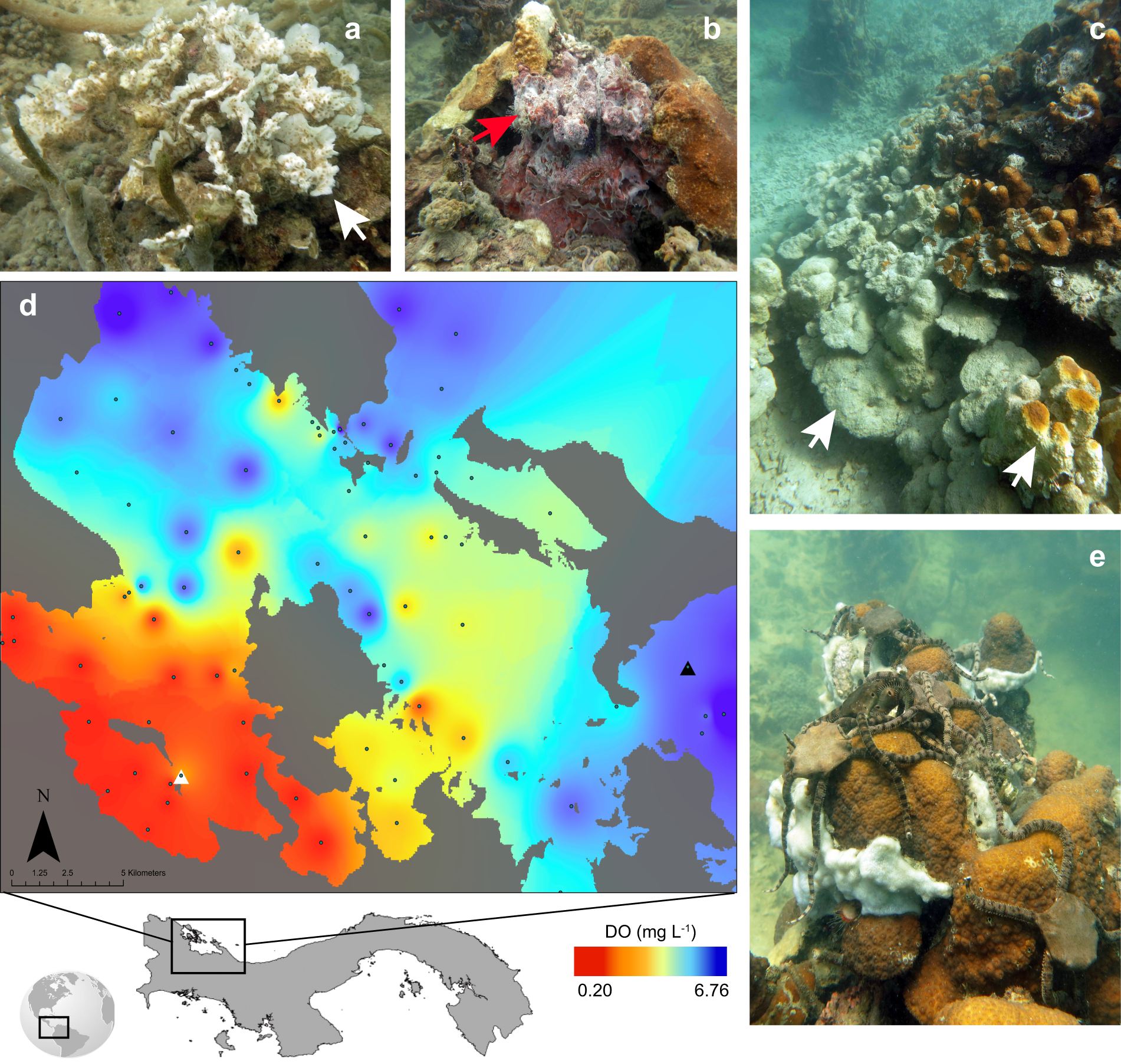The image collage, comprising five labeled sections (A, B, C, D, and E), predominantly showcases underwater coral formations, with a single map image. Each coral photograph (A, B, C, and E) is highlighted with arrows indicating specific areas, likely where coral bleaching is occurring, attributed to rising water temperatures. Image A depicts a predominantly white, bleached coral. Image B features a coral with a pinkish-red hue, while Image C displays both live and bleached corals. Image E stands out with various octopuses sitting atop the coral, which also shows significant bleaching. Image D diverges from the coral photographs, presenting a color-coded map that identifies sea temperatures, ranging from hotter regions in red to cooler regions in blue, with additional color gradations in purple, yellow, orange, and green. This map, featuring labels and a scale indicating distances in kilometers, suggests regions affected by temperature variations that could impact coral health. The comprehensive visual narrative underscores the detrimental effects of temperature changes on coral reefs through a combination of detailed photographs and a supporting temperature distribution map.